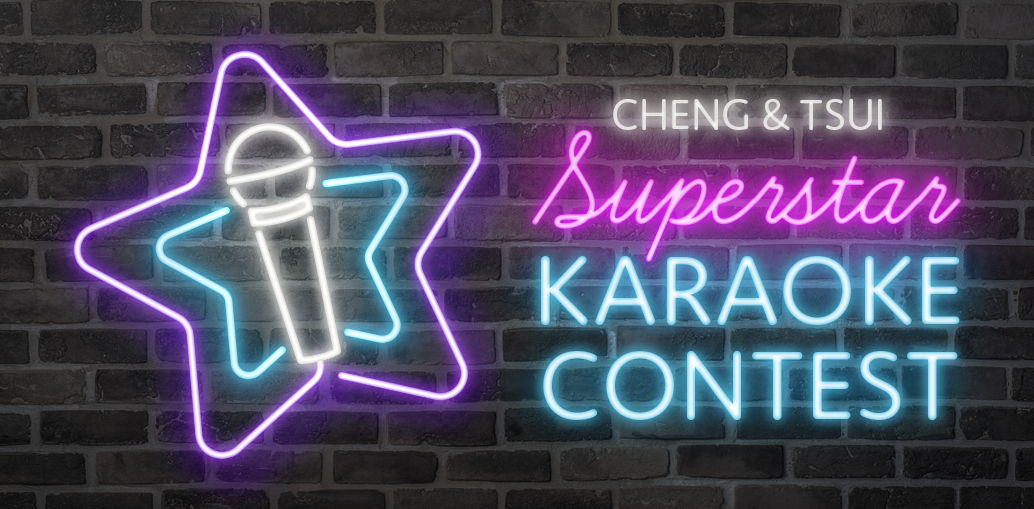The image depicts a digitally composed neon sign displayed on a horizontally-aligned grayscale brick wall with alternating black and gray bricks and gray grout in between the bricks. On the left side of the sign, there is an illuminated purple star outline, within which there is a smaller blue star outline and a white neon microphone at the center. Adjacent to this, on the right side, is a series of neon-lit words, each centered sequentially. The first line reads "Chang & Tsui" in white light, followed by the word "Superstar" in cursive purple neon, and finally, "KARAOKE CONTEST" in all capital letters, presented in light whitish-blue neon. The entire composition of neon elements contrasts vividly against the brick backdrop, promoting the "Chang & Tsui Superstar Karaoke Contest."